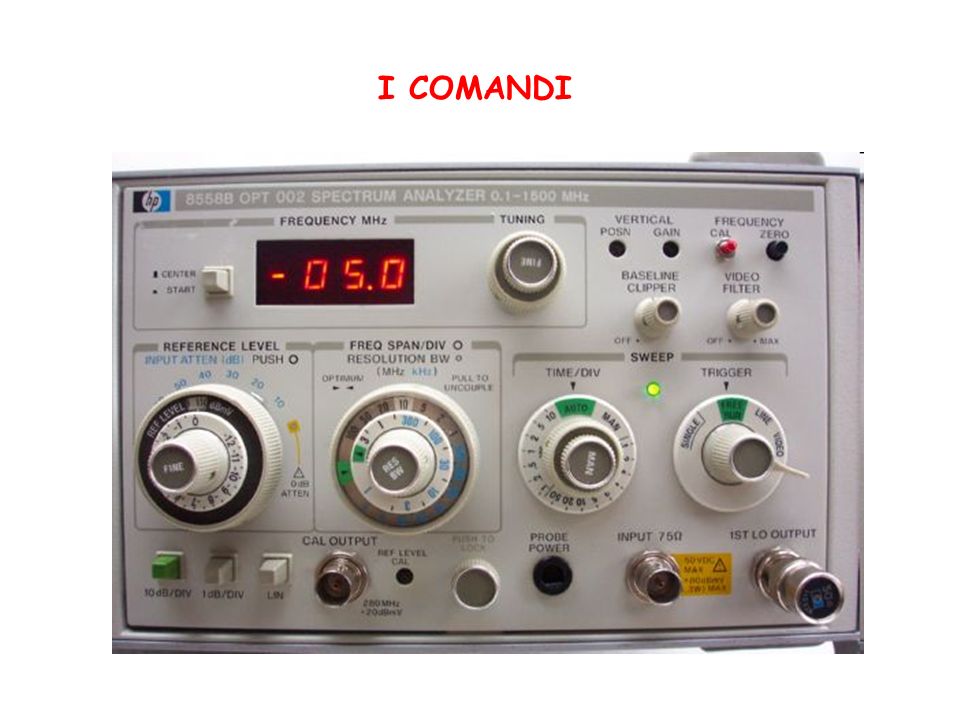This image depicts an HP 85588 OPT-002 Spectrum Analyzer, an electronic device characterized by its predominantly white and gray body with various red elements. The top of the device features the text "ICOMANDY" in bold, red, capital letters set against a white background. Below this, the analyzer displays a small LED screen indicating a frequency measurement of "-0.5 MHz" in bright red digital numerals. 

The interface of the spectrum analyzer is populated with numerous knobs and buttons, each designated for specific functions such as tuning, vertical frequency, baseline, and video filtering. Notably, there are adjustments for reference level, frequency span, time division, and trigger, along with input and output ports, including the "Cal Output" switch and "Probe Power" and "Input 75 Omega" jacks. The detailed configuration options, including the frequency, gain, and sweep dials, highlight the device's intricate design tailored for precise electronic measurements.